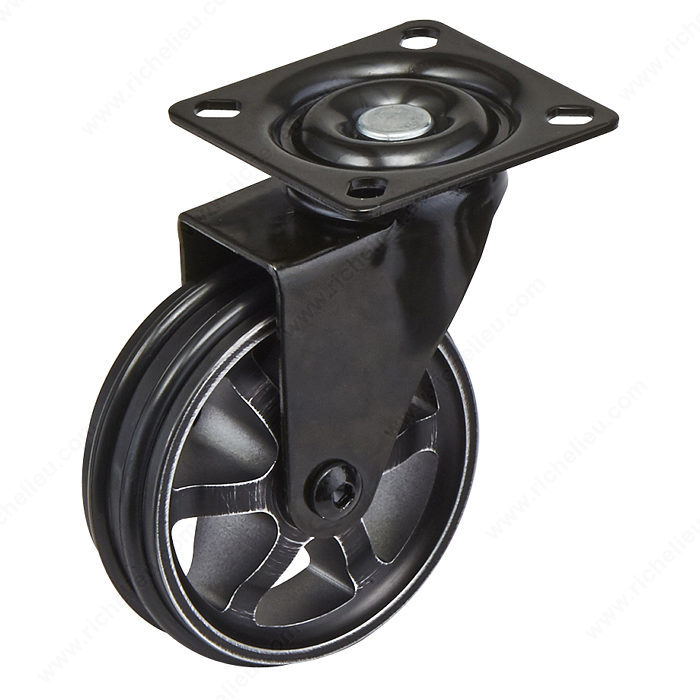This close-up, angled, photorealistic image showcases a small black metal wheel, devoid of a rubber tire, set against a pure white background. The wheel features two grooves in its center and is secured by a black screw that runs through its midsection. A black bracket, held firmly by this screw, is attached to the wheel. Atop this bracket is a square metal plate with a silver center and a black surrounding "donut" section. This flat plate includes four oval openings, evenly distributed with two on the top and two on the bottom, designed to allow the attachment of additional components. The wheel, slightly worn with visible scratches revealing the underlying silver metal, sports five spokes and is positioned at the bottom of the image. The overall perspective is slanted downwards from a bird's eye view, emphasizing a sense of suspension within the white void, reminiscent of clipart. This configuration suggests versatility for various applications, such as being mounted onto a trolley or other equipment to enhance mobility.